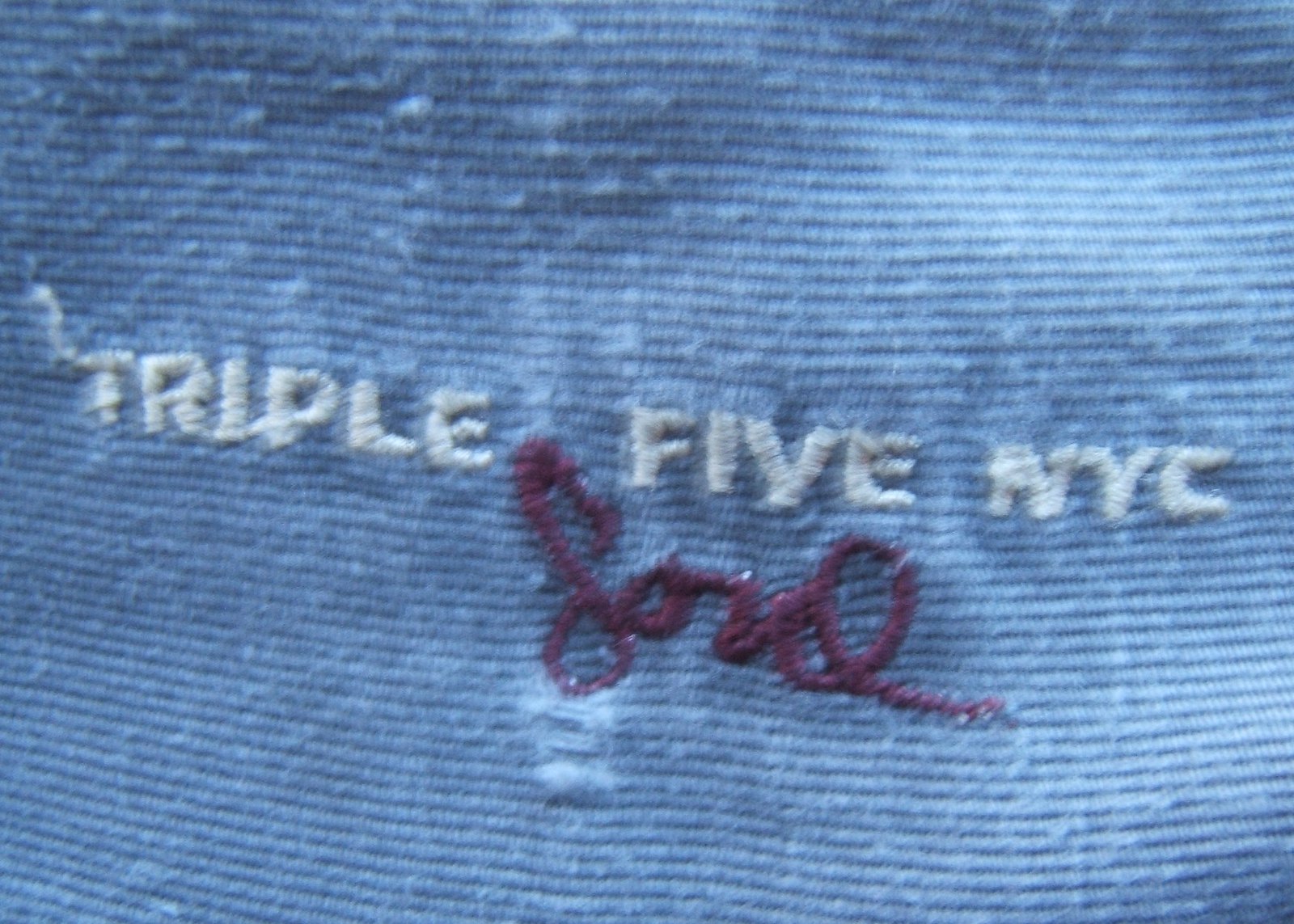The image shows an up-close view of a blue fabric, possibly from a pair of jeans, a jacket, or a work shirt. The material appears slightly worn with visible fiber pills and a few frayed and raised areas, particularly in the top right-hand corner where the fabric looks more faded, almost whitish-blue. Embroidered in white capital letters is the text "TRIPLE 5 NYC," while in cursive maroon stitching below the word "FIVE," the word "SOUL" can be seen. The background fabric, with its varying shades and wear, suggests heavy usage or vintage quality. No other identifiable features such as pockets or tags are visible.